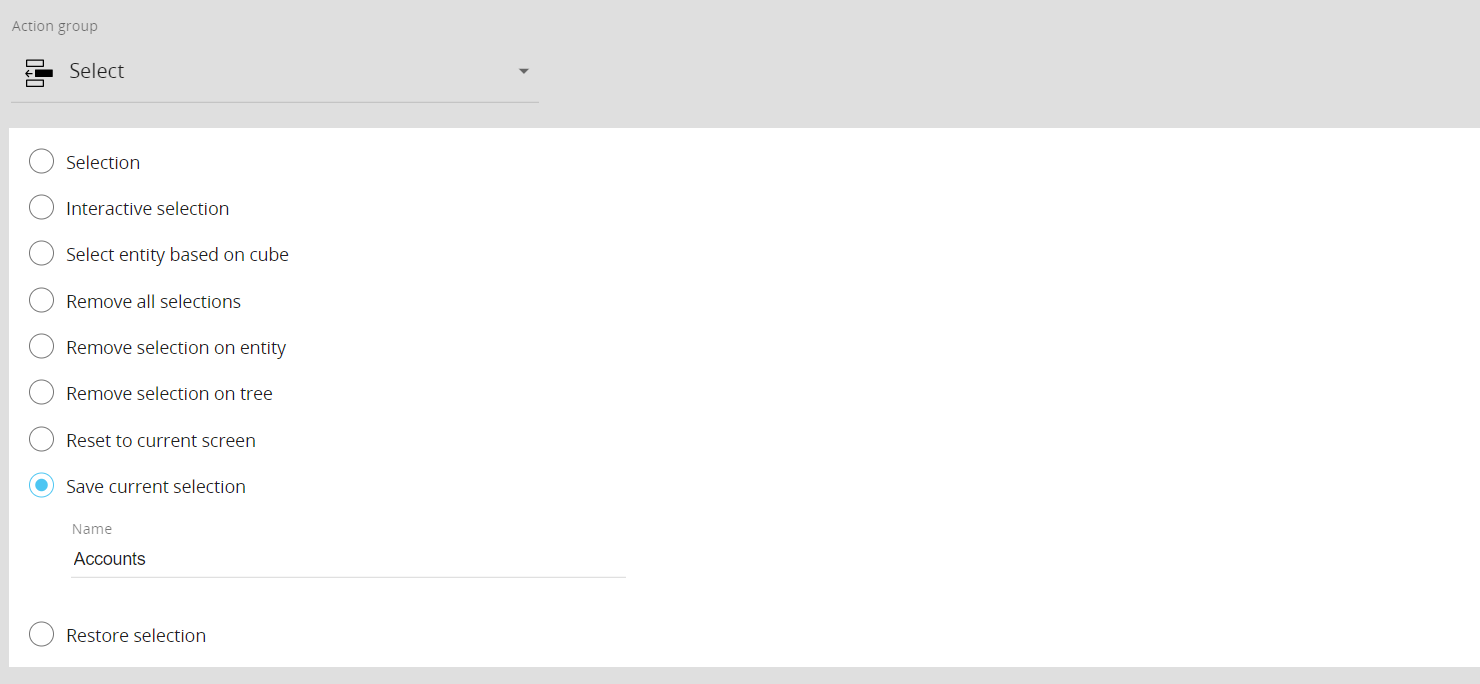The image appears to be a screenshot of a website's filtering page. At the top of the page, there is a heading labeled "Action Group." Directly below this heading, there are a series of clickable buttons organized in a vertical list. The first button is labeled "Selection," followed by "Interactive Selection," "Select Entity Based on Queue," "Remove All Selections," "Remove Selections on Entity," "Remove Selection on Tree," "Reset Root Screen," and "Save Current Selection," which is currently activated as indicated by a blue-filled circle to its left. The label next to it reads "Name Accounts." The final button in the list is labeled "Restore Selection."